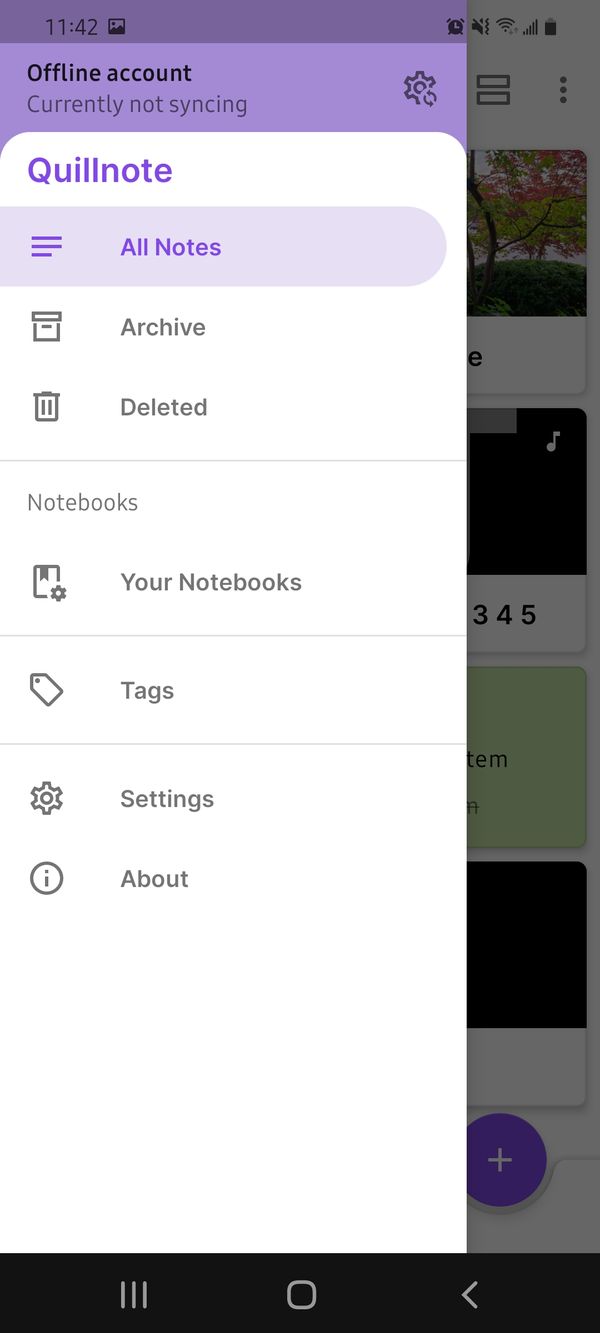This image depicts a sidebar from a webpage. The sidebar is divided into two distinct color sections. The top portion is lilac purple, featuring the following elements from top to bottom: the time "11:42" at the upper-left corner, a picture icon, and the text "Offline - Account Currently Not Syncing" with a gear icon to its right. 

Below this lilac purple section, the rest of the sidebar is white. At the top of the white section, there's a line of text "Quill Note" in purple. Directly beneath this, there are three menu options arranged in rows: "All Notes" (highlighted in purple to indicate active selection), "Archive," and "Delete". Next, the second section labeled "Notebooks" follows with four options: "Your Notebooks," "Tags," "Settings," and "About." Each option is accompanied by a corresponding icon to the left of the text: a notebook icon for "Your Notebooks," a price tag for "Tags," a gear for "Settings," and an information symbol for "About." Similarly, the "Delete" option has a trash can icon, and "Archive" is represented by a box icon.

At the very bottom of the sidebar is a black stripe, but its contents are not described. The webpage behind the sidebar is grayed out and appears to contain approximately four or five sections.